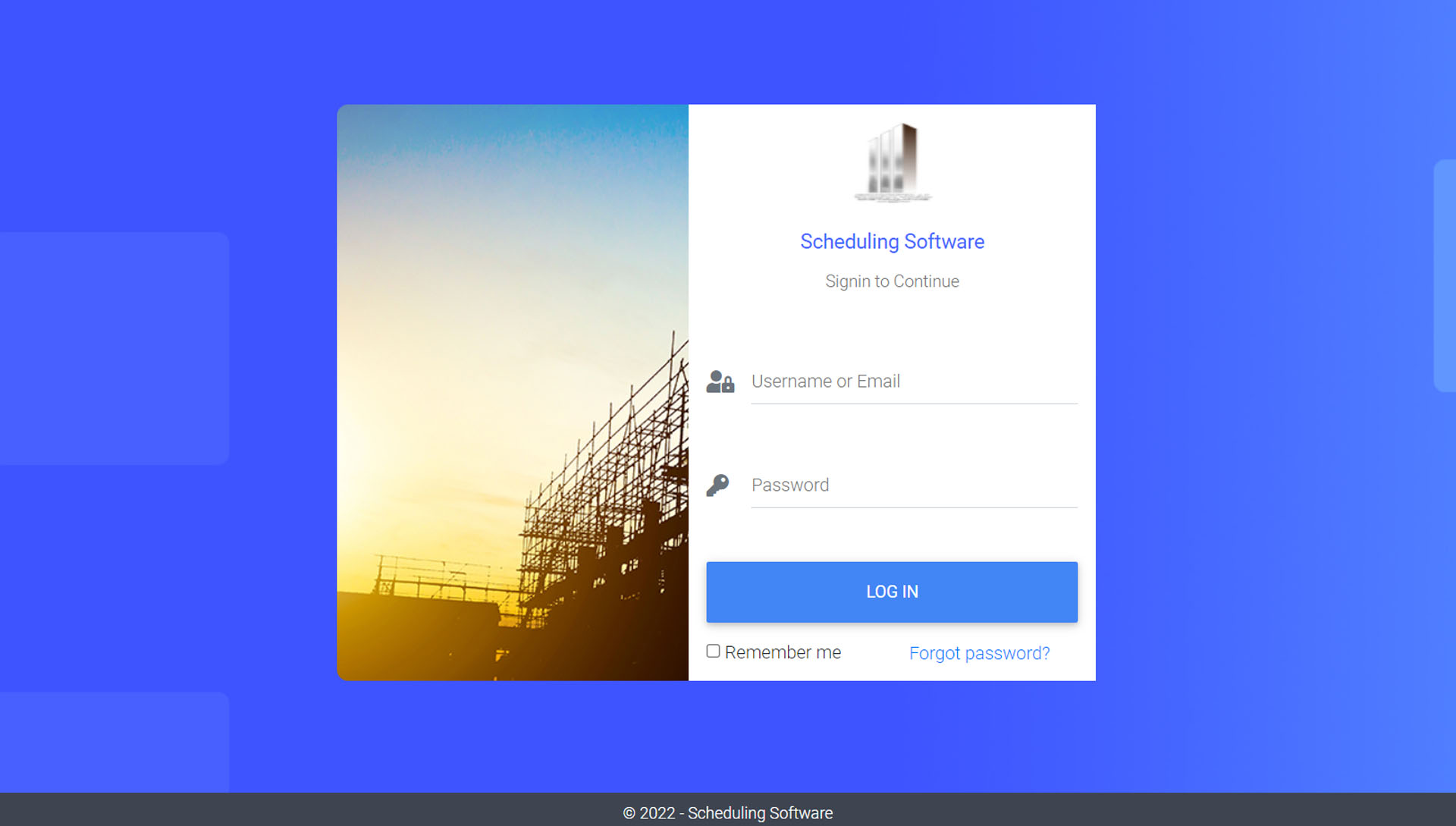The image depicts a computer login screen with a dynamic blue background composed of varying shades, transitioning from darker in the top left corner to lighter in the bottom right. The background is punctuated by several gently floating, lighter blue squares, adding a modern aesthetic touch.

Centrally positioned on the screen is the main login interface, divided into two sections. The left section, slightly less than half the width of the interface, features a photograph likely taken at either sunrise or sunset. This photograph captures what appears to be a construction site at the bottom, with a gradient sky transitioning from a warm yellow near the horizon to a serene blue at the top, suggesting the onset or conclusion of the day.

The right section of the interface highlights the login functionalities. At the top, there is a symbol resembling a building, followed by the text "Scheduling Software" in blue. Below this, it instructs users to "Sign in to Continue" in grey. There is a graphical silhouette of a person with a padlock icon beside a text box, designated for entering the username or email. Directly beneath is another text box, this one preceded by a key icon and labeled "Password."

At the bottom of this section is a prominent blue button with white text reading "Log in." Below this button is a checkbox for "Remember me," and to the right, a clickable blue link that reads "Forgot password."

Spanning the entire width at the bottom of the screen is a thin, dark grey bar. Centrally placed within this bar, the text "Copyright 2022-Scheduling Software" is displayed in white, providing legal and ownership information.